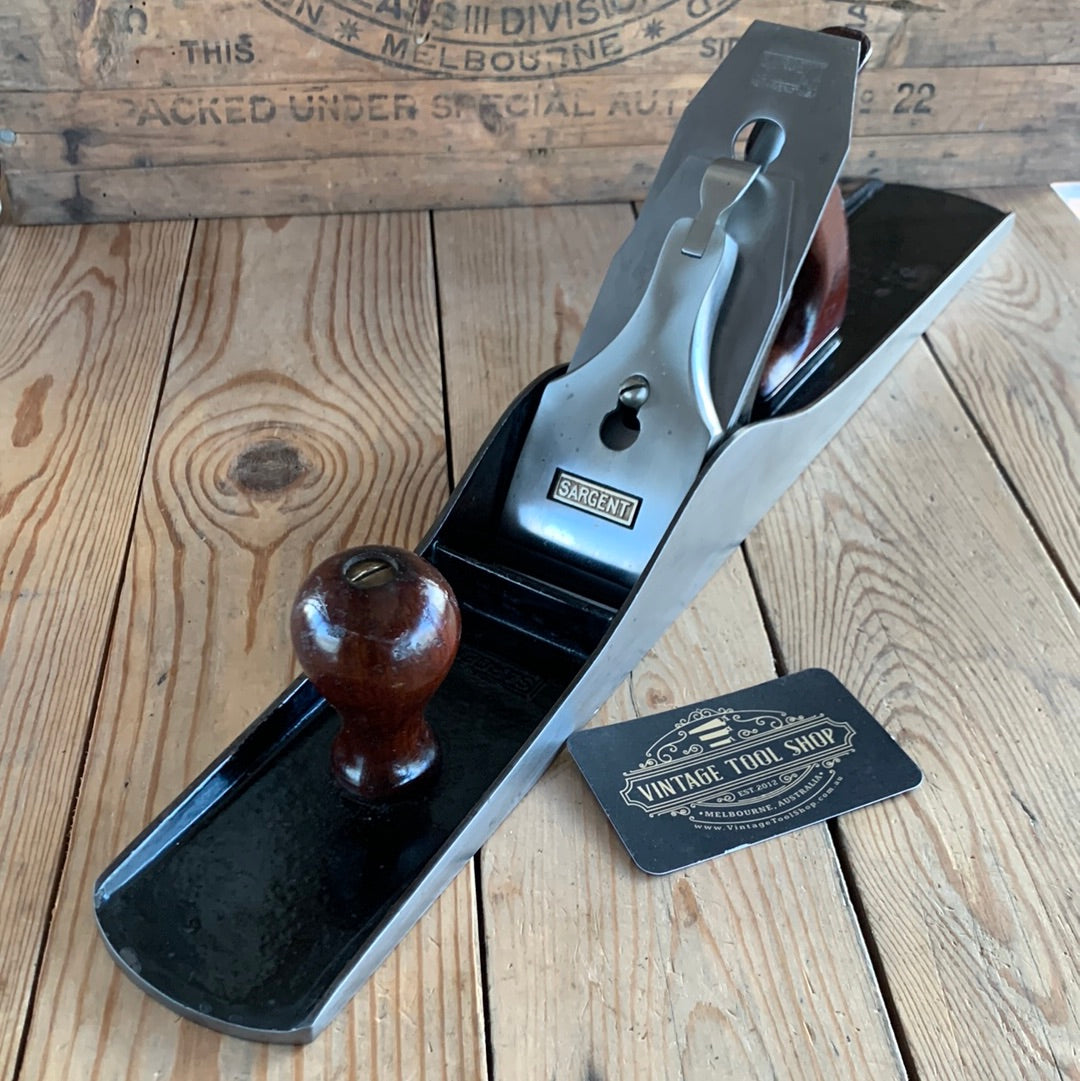The image showcases a vintage metal tool, most likely a wood planer, situated on a wooden deck table or bench. The background features a wooden box stamped with the partially visible text, "Packed under special authority number 22 Melbourne." In front of the tool lies a small leather patch emblazoned with "Vintage Tool Shop Melbourne Australia" and a stylized logo. The tool itself bears the brand name "Sargent" and appears to have a dual-handle design—one wooden handle at the back and another integral handle at the front. The tool's construction and design, including its diagonal metal piece, suggest its primary function is for cleaning or planing wood.